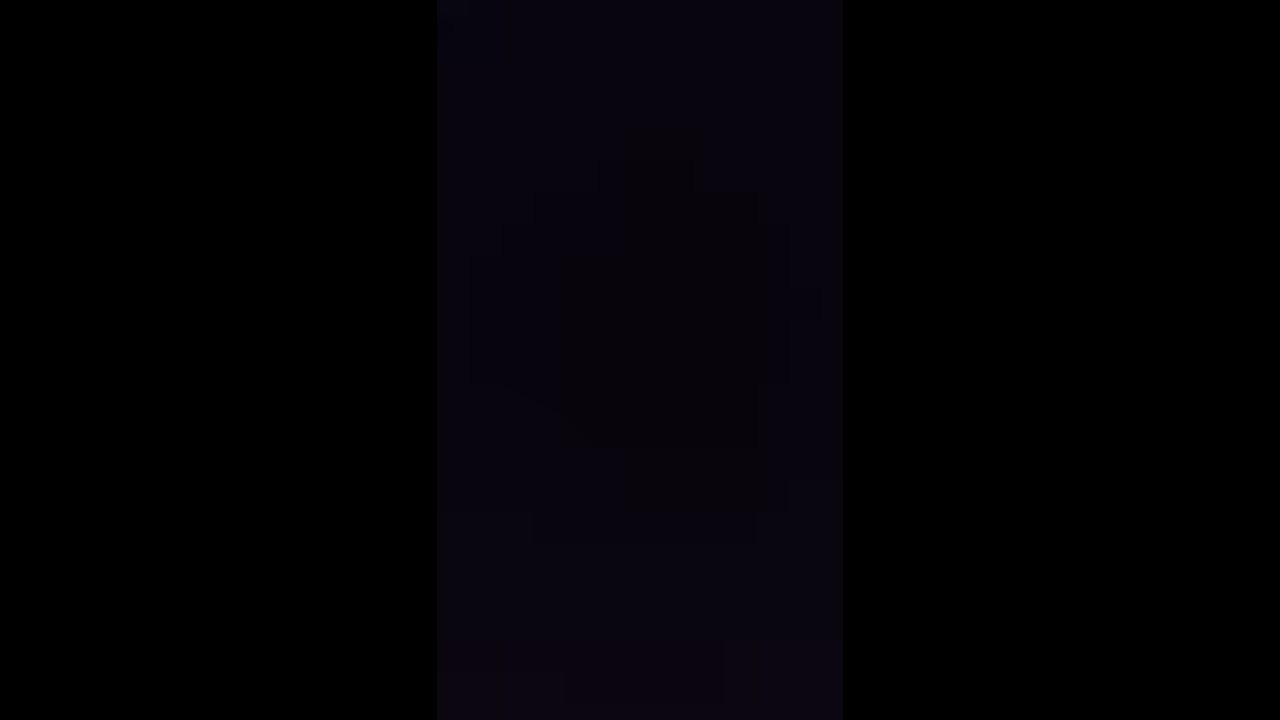This image features a solid black rectangular background that appears entirely devoid of any notable objects or features at first glance. The rectangle spans approximately 6 inches in width and 3.5 inches in height. Yet, upon closer inspection, subtle variations in shade become evident. The far left and far right sections are a deep, rich black, occasionally noted to have a slightly reddish hue—indicative of a true, intense black color. The center strip, occupying a little over a quarter but less than half of the width of the image, exhibits a very dark navy blue tint with a faded, hazy, bluish-black appearance, as if emanating from a computer screen. This central section has a barely perceptible darker black spot, which may appear different depending on the viewing angle, sometimes resembling a backward "D" or a segment of a circle. The absence of any frame, text, icons, or graphics draws attention to these understated differences in color, making this seemingly plain jet-black image intriguing in its subtle complexity.